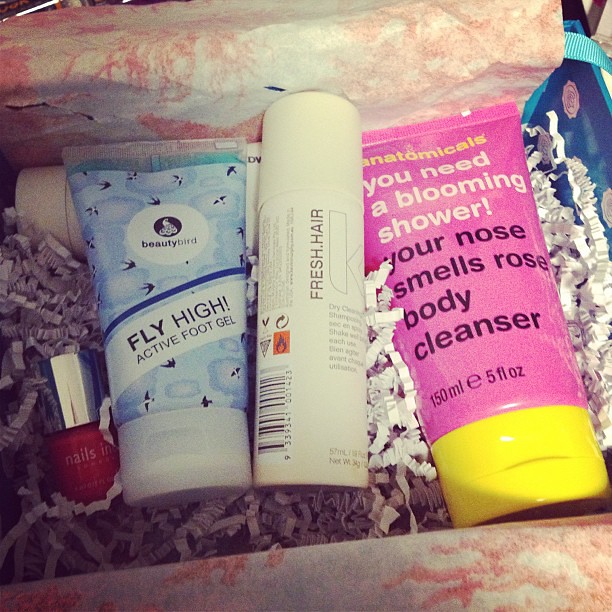The image is a color photograph in a square format, capturing a box filled with various beauty and hygiene products nestled in stringy crinkled white paper and marbled peach and white paper. On the right side, there is a prominent pink squeeze bottle with a blue cap, labeled “anatomicals: you need a blooming shower, your nose smells rose, body cleanser, 150ml, E5-FLOZ.” In the middle, a white bottle with black vertical text reads "fresh air," and it features a slightly darker white cap. To the left of this, a light blue and white squeeze bottle adorned with darker blue circles and birds is marked with "beauty bird" in a central white circle and "fly high active foot gel" diagonally below it. At the bottom left, a small nail polish bottle with a silver cap sits alongside the other products. The box’s edge reveals a partial blue section with an aqua-blue ribbon. The image exemplifies photographic realism in product photography, showcasing a neatly arranged collection of grooming items.